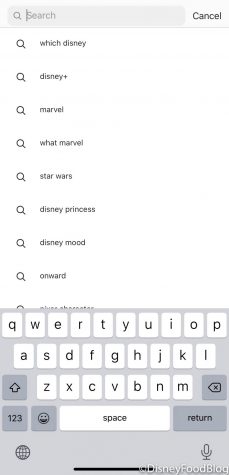A person is performing a search on their iPhone. At the top of the screen, a rectangular search bar with very rounded corners sits against a header that is an even lighter shade of gray than the bar itself. On the left side of the search bar, there is a medium gray magnifying glass icon, followed by a blinking gray cursor. To the right, in light gray lettering, the word "Search" is visible. Further to the right, the word "Cancel" appears in black lettering.

Beneath the search bar, multiple search suggestions are listed in small black text, each preceded by a small dark gray magnifying glass icon. The suggestions include: "which Disney?", "Disney plus", "Marvel", "what Marvel", "star Wars", "Disney princess", "Disney mood", and "Onward." A final suggestion is present but gets cut off.

Below the search suggestions, the iPhone's traditional QWERTY keyboard is displayed. The keys have a medium gray background, while the letter keys themselves are white with black sans-serif lettering. Certain function keys, including the shift (uppercase) key, the "123" key, the emoji key, the return key, and the backspace key, possess darker gray backgrounds but maintain the same black text. On the bottom left corner of the keyboard, a dark gray globe icon is visible, and on the bottom right, there is a gray microphone icon.

Near the bottom-right corner of the screen, a tag reads "© Disney Food Blog" in white text, accompanied by a white copyright symbol.